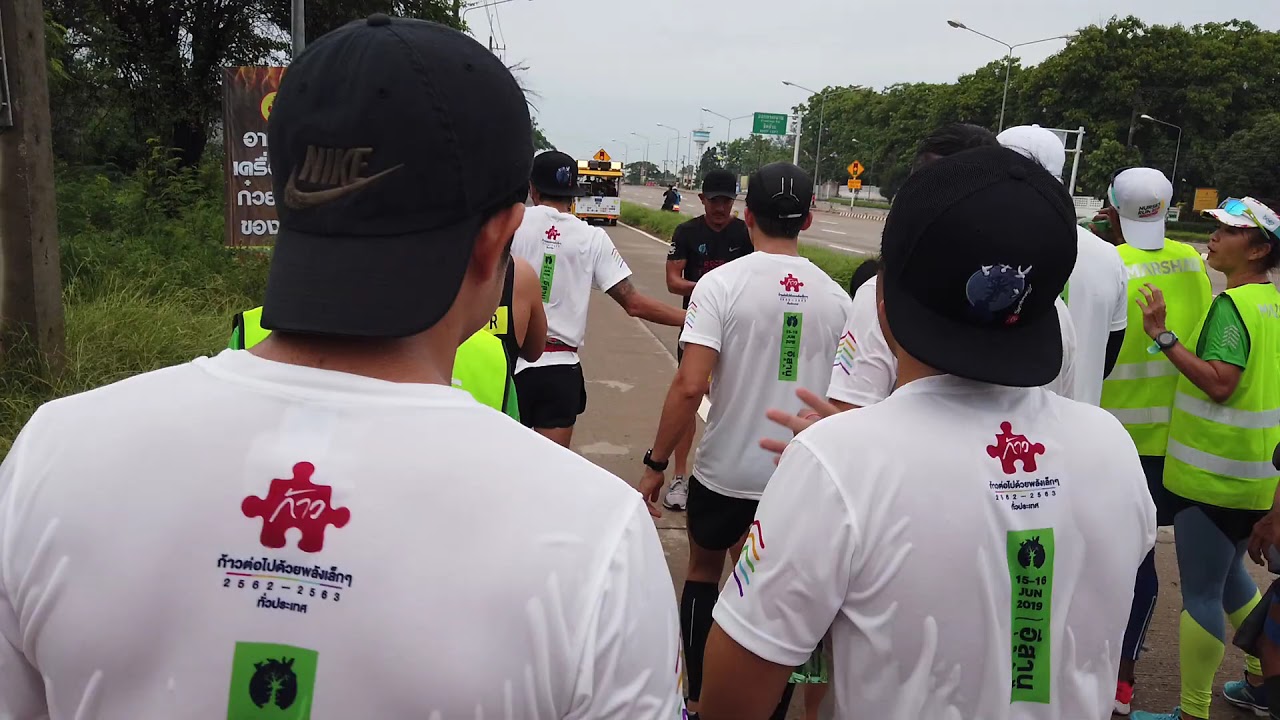This daytime outdoor photograph captures what appears to be a charity or athletic event, possibly a running or walking marathon. A large group of participants, all wearing the same white T-shirts with black shorts, are visible from behind. Leading the group in the foreground are two men in black baseball caps, turned backwards, showcasing the event’s uniform. Their shirts display a red puzzle piece logo below which is a series of text in an Asian language, possibly Thai, and dates reading "15th to 16th of June 2019." Below the text is a green rectangular design. Additional runners, also in white T-shirts and backwards caps, are visible ahead of them. High-visibility marshals, sporting neon vests marked "Marshall", and some wearing caps or visors, are interspersed among the participants. Notably, a woman in yellow high-vis attire and blue-and-yellow tights stands out in the crowd. Facing the group from a distance, a man dressed in black appears to be coordinating the event. The scene is set against a backdrop of a road extending into the distance, lined with trees on both sides and featuring overhead streetlights, signs, and road markings, indicating a major roadway or highway. Vehicles, including a moped, can be seen on the road, contributing to the lively atmosphere of the event.